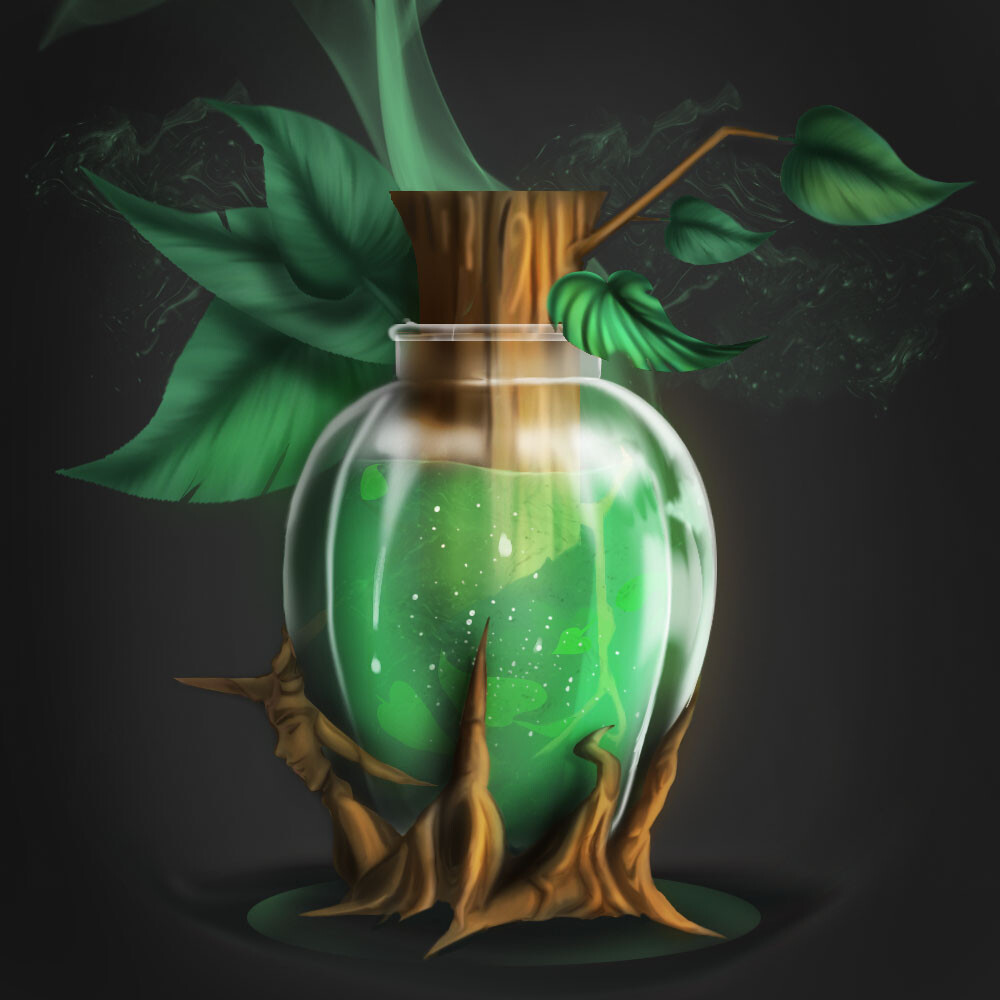The image is a detailed computer-generated artwork showcasing a clear glass vase with a distinct, curved, oval shape. The vase contains a light green liquid, emphasizing its glassy texture with visible white highlights. Emerging from the liquid is a gold-colored, gnarled branch that protrudes through the top of the vase, featuring three green leaves on a smaller branch. The branch has an eerie carved face resembling a helmet or headdress on the bottom left side. The base of the vase incorporates brown wood elements, giving an organic contrast to the clear glass. At the top, the vase is sealed with a natural wood cork, from which green, cloudy smoke appears to be emanating. The whole composition is set against a dark gray, almost black background, adding a dramatic ambiance to the scene.